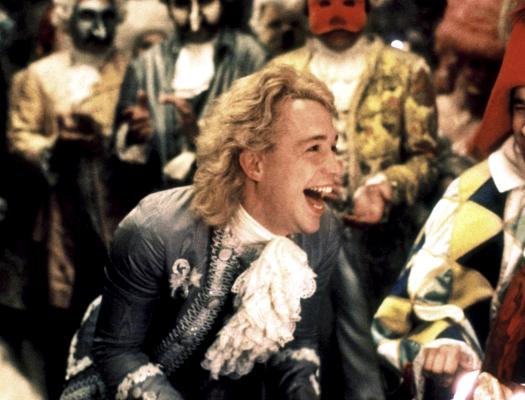This is a close-up, grainy photograph of a man with shoulder-length, wavy blonde hair, captured mid-laugh, clearly enjoying himself. He is slightly crouched with his hands extended forward and down, almost as if he were playing an invisible piano. His attire is distinctive and old-fashioned, featuring a long gray leather jacket adorned with white frills or a poofy scarf. The scene behind him is blurred, revealing a gathering of people in elaborate costumes and masks, suggestive of a masquerade ball. Noteworthy among them is an individual to his left dressed as a court jester in a colorful costume with a red hat. The overall setting evokes a lively and whimsical atmosphere, with the man at the center having the time of his life.